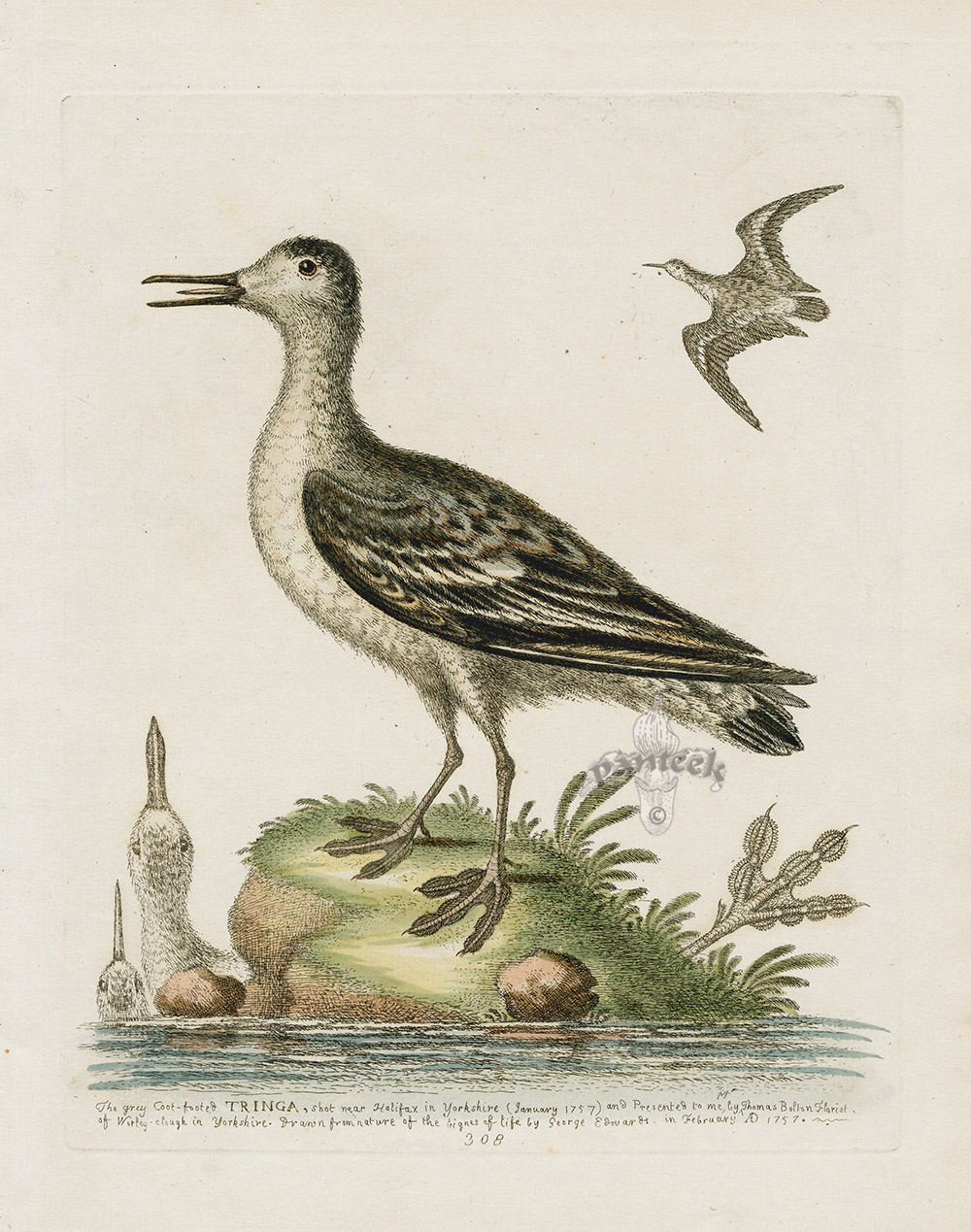This intricately detailed image appears to be a vintage colored pencil drawing of a bird, likely a species within the genus "Tringa." The bird is perched on a small, grassy and rocky island surrounded by water. The vivid scene is minimally colored, showcasing muted tones with a hint of green on the grass and various shades of brown on the ground. The bird itself features a black beak, a black crown that extends down its back, and black, tan, and white stripes on its wings. Beneath the adult bird are two juvenile birds, their beaks pointing straight up and their heads similarly colored in hues of white and black. In the background, another bird, resembling the one perched on the island, is depicted flying through the sky. The overall image, including the finely detailed line art, is very aged, adding a yellowish tint across the page, indicative of its vintage nature. The scene is part of a book illustration, as suggested by the presence of a visible page and a watermark labeled "Pantique" on the right side. Below the image is some small, fine handwriting, possibly identifying the bird species, but the text is largely unreadable. The visual composition is minimal, with the isolated island and a single bird in flight providing the only background elements.